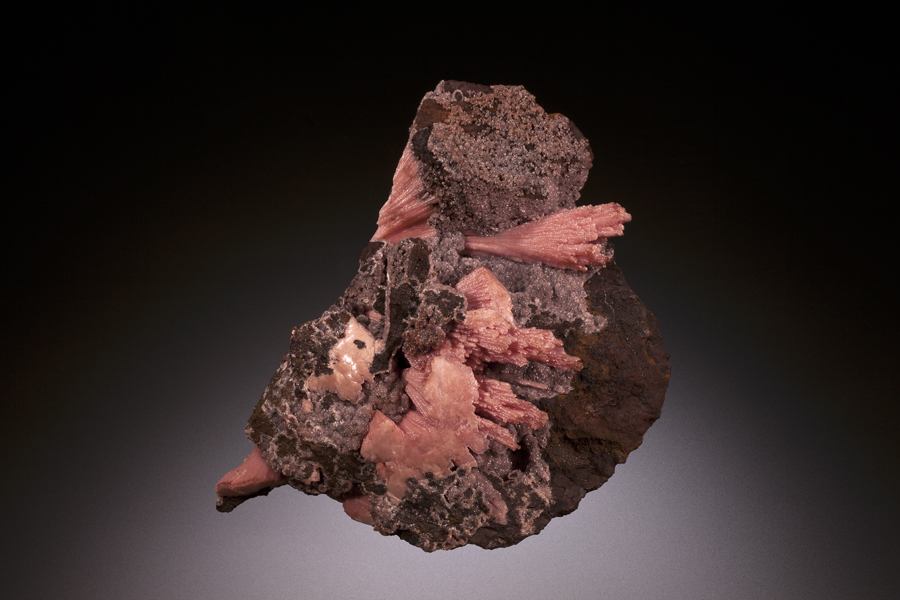The photograph features a distinctive rock prominently displayed in the center against a gradated black-and-white background, which transitions from white beneath the rock to darker shades of gray towards the edges, notably darker in the top right and left corners. The rock is multifaceted with a mixture of browns, reds, and hints of pink, resembling a human heart in shape. The rock's base is a dark chocolate brown, particularly noticeable in the bottom right corner. Interspersed within its solid mass are brighter red crystal formations, suggesting an iron-rich composition possibly akin to rhodochrosite, with salmon-colored, fiber-like strands emerging from the structure reminiscent of thin wires or fiber optic cables. Additionally, there's a small, shiny white segment located on the lower left corner. The rock's unique combination of colors and textures, including pinkish tissue-like areas and spongy brown patches, lends it an organic appearance that could be likened to an internal organ or an underwater coral formation. The lighting highlights the rock's varied surface, making each nuanced detail visible and vivid amidst a somewhat blurry background.